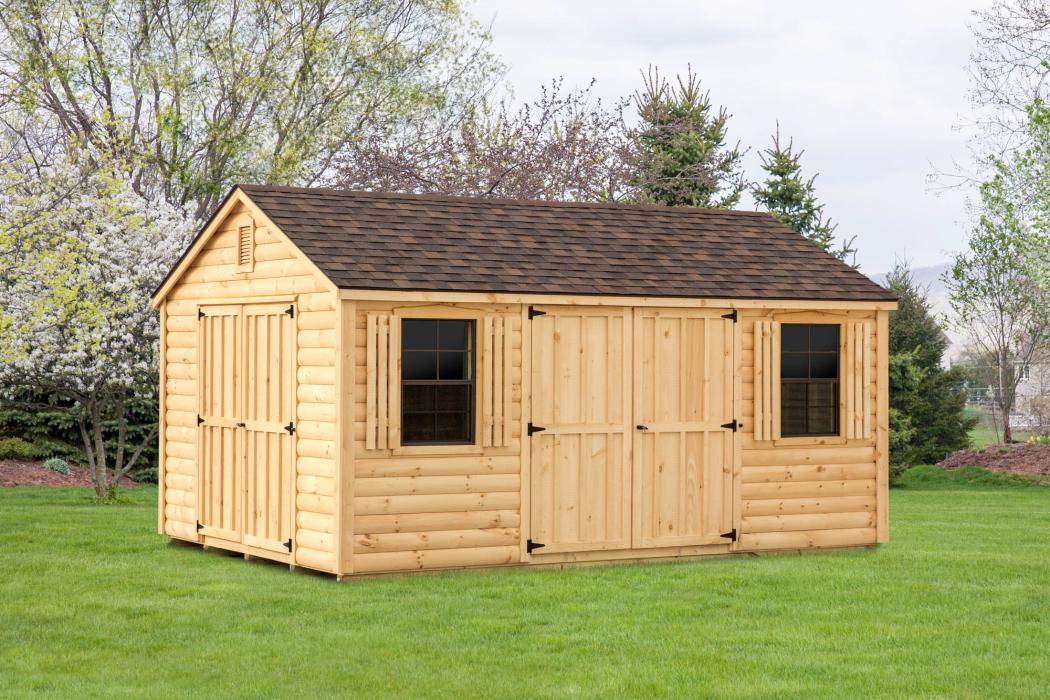This image showcases a well-crafted, unfinished wooden storage shed, prominently centered in an immaculate, well-maintained backyard. The shed features light brown wood panels and posts, reminiscent of pine wood, and is capped with a grayish brown asphalt shingle roof, likely a single layer. Two wooden doors with black metal shed hinges and a central black handle open from the middle, flanked by windows on either side, adorned with wooden shutters. Above the doors is a wood louver roof vent providing ventilation.

The shed is surrounded by freshly cut green grass that contrasts with the carefully placed small trees and bushes in the background. Behind the shed, trees with green leaves and white flowers rise against a partly cloudy sky, creating a serene, picturesque setting. The overall scene exudes a sense of meticulous care and peaceful outdoor charm, likely someone's cherished backyard.